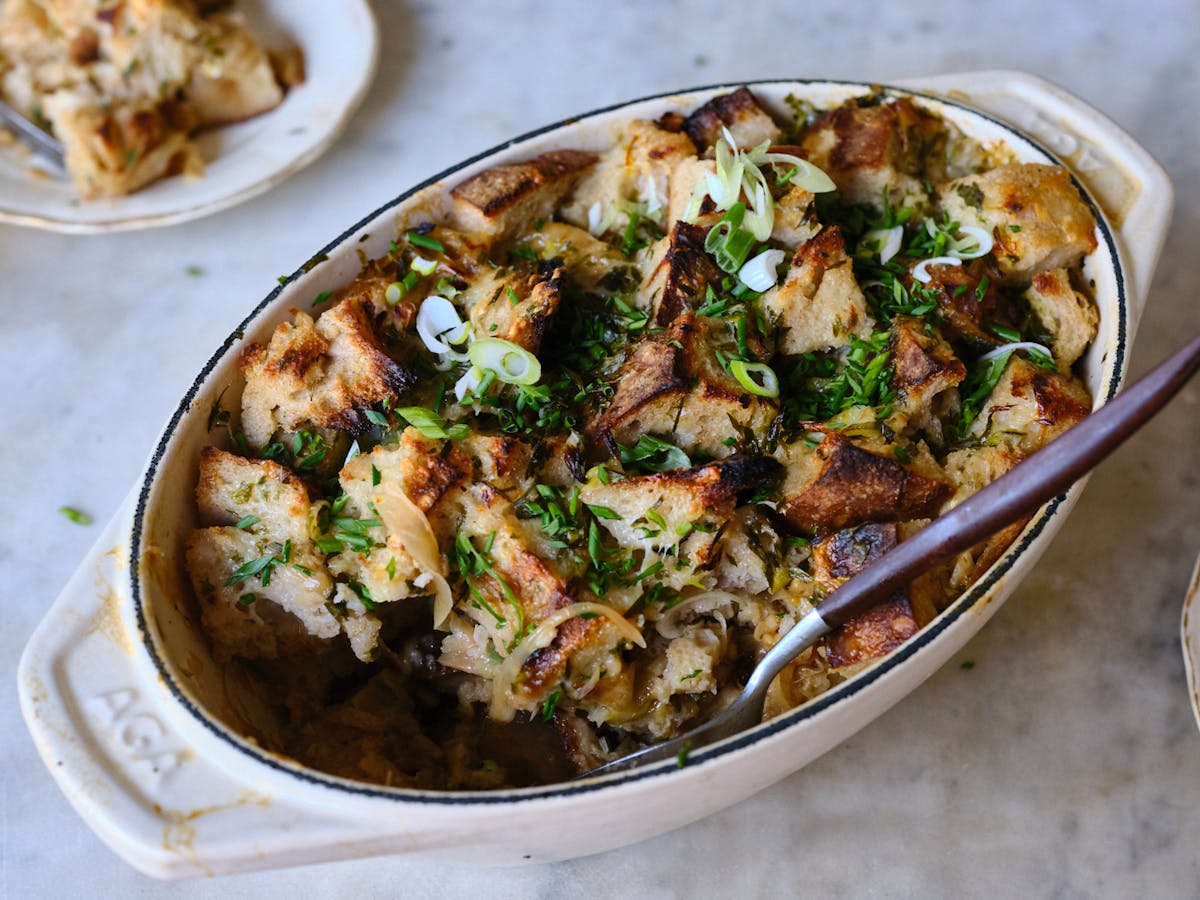The color photograph captures a white, oval-shaped, metallic bowl with small handles on both sides, each inscribed with the letters "AGA." The bowl, which features a distinctive black rim, is filled with what appears to be cooked and cut-up chicken, browned on top, and adorned with various green herbs such as green onions, basil, and parsley. Grilled onions and scallions are also visible among the ingredients. Resting inside the bowl is a spoon with a wooden handle and a metallic end. On the upper left corner of the image, there is another plate containing some of the same meat with a fork in it, while a partial view of an additional plate is visible on the right. The marble table beneath the dishes complements the overall presentation, with its white and black veining adding to the detail and clarity of the setting.